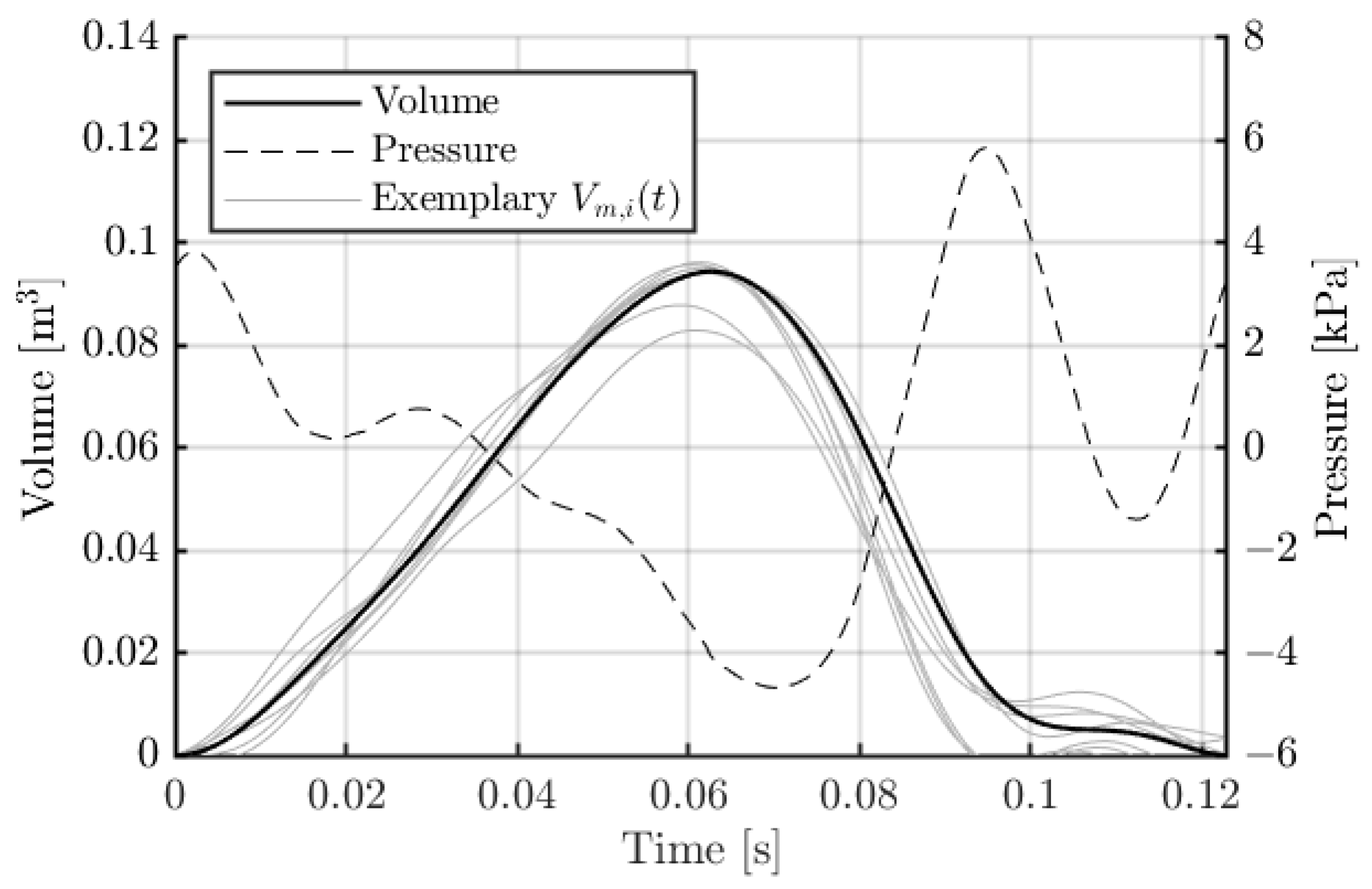The graph illustrates the relationships between volume, pressure, and time in a scientific context, displayed in a landscape orientation and depicted in black and white. The horizontal X-axis represents time in seconds, ranging from 0.00 to 0.12. The vertical Y-axis on the left shows volume in cubic meters (m³), with increments from 0 to 0.14. A secondary Y-axis on the right indicates pressure in kilopascals (kPa), scaling from -6 to 8.

Three distinct lines are plotted:
1. A solid black line representing volume.
2. A dashed line indicating pressure.
3. A light gray line marked as "exemplary VMI(T)."

The graph features grid markings and includes a legend in the top left corner for clarity. The volume line starts low, peaks at the center, and then descends. The pressure line exhibits more erratic fluctuations. This visual representation helps illustrate the dynamic interplay between volume and pressure over time.